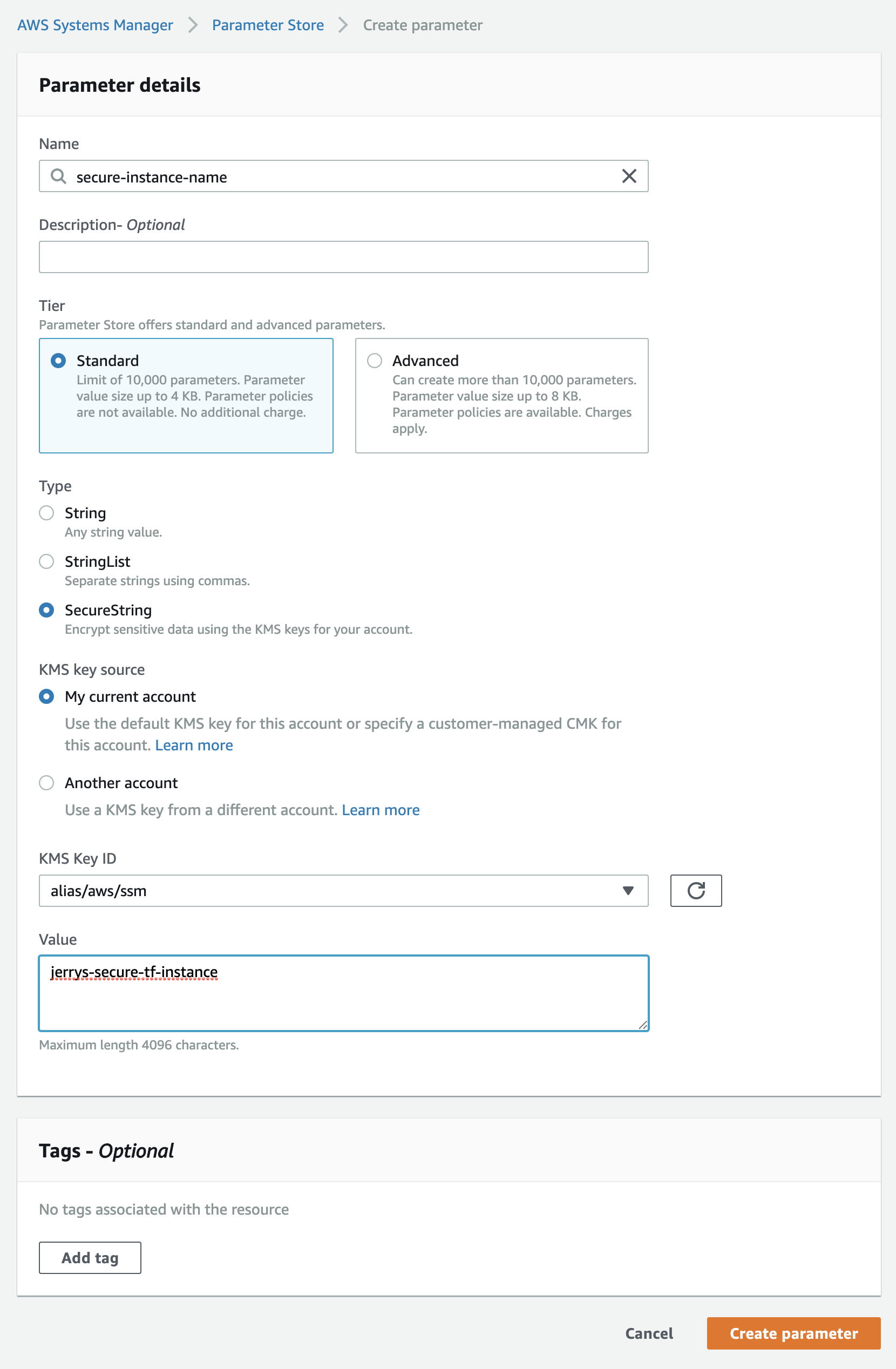Here is an improved and detailed caption based on the provided description:

---

Screenshot of a section from a web management interface on the AWS Systems Manager Console. The breadcrumb navigation at the top indicates the user navigated from "AWS Systems Manager" to "Parameter Store" and finally to "Create Parameter," suggesting that a new parameter is being created.

The main content area is titled "Parameter Details." Within this section:

- "Name": The user has entered "Secure Instance Name."
- "Description": No information has been entered yet.
- "Tier": The user has selected the "Standard" tier, which supports up to 10,000 parameters, with each parameter value being no more than 4 kilobytes. Note that 'Parameter policies' are not available in this tier and there is no additional charge.
- "Type": The user has chosen "Secure String," intended for encrypting sensitive data using AWS Key Management Service (KMS) keys.
- "KMS Key Source": The user opted for "My Current Account," indicating that the KMS key used for encryption is managed within the current AWS account.
- "KMS Key ID": The entry here is "alias/aws/ssm."
- "Value": The value set is "Jerry Secure TF Instance."
- "Tags": No tags have been added yet.

This detailed setup aids in securely managing configuration data and secrets necessary for deployments and operations.